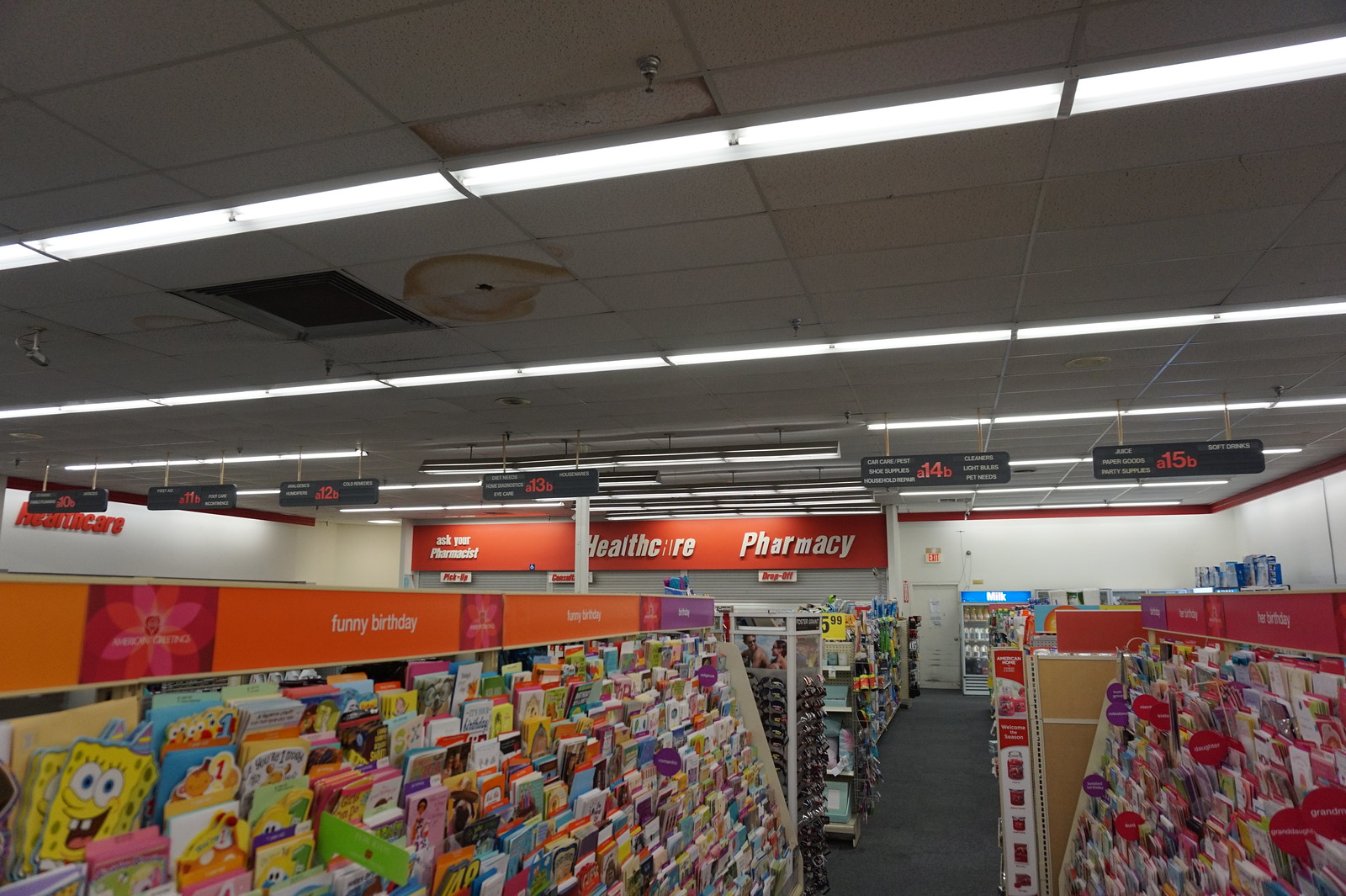This photograph captures the interior of a small pharmacy, reminiscent of a CVS or dollar store, with a scene centered around greeting cards. At the front of the store, there is a card rack prominently labeled "Funny Birthday," showcasing a variety of cards, including eye-catching Spongebob-themed cards on the left-hand side, while more adult-oriented cards are on the right. The aisle signs are clearly marked, with row indicators and product listings, such as "Row 14B: Car Care Cleaners, Light Bulbs." The store features gray carpet flooring and open fridges with drinks against the far wall. Towards the back of the store, under red trim above white walls, is a shuttered section labeled "Health Care Pharmacy" and "Astro Pharmacist," indicating that the pharmacy counter is currently closed. Additionally, there is a rotating sunglasses display near the card section, adding to the diverse offerings of this compact, neighborhood-focused store.